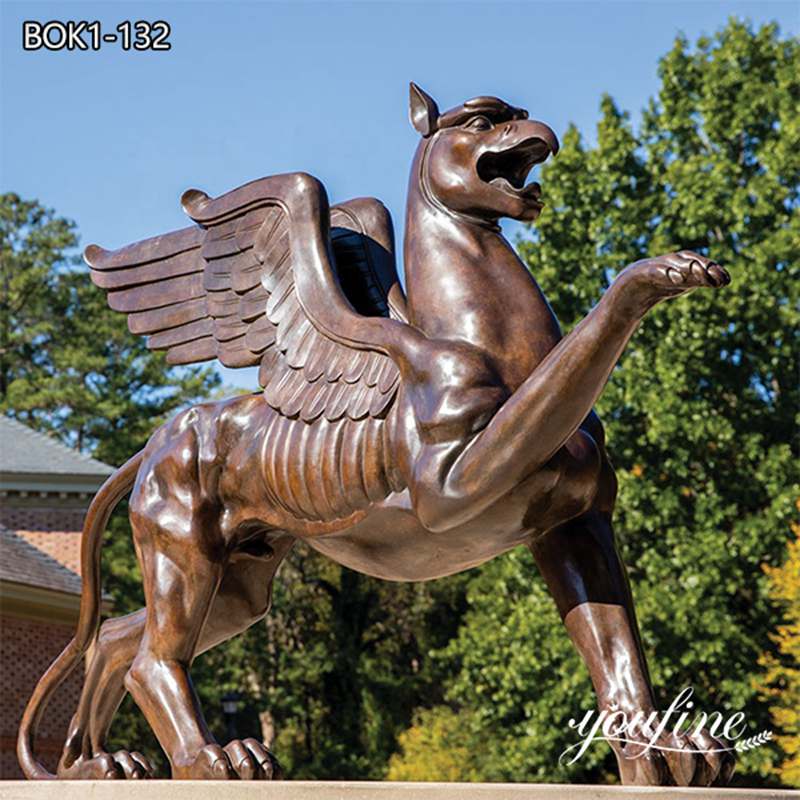The photograph depicts a very large bronze statue of a griffin set outdoors against a background of trees and a vibrant blue sky. The griffin, a mythical creature, features prominent wings, a long tail, and one of its front paws raised as if ready to strike. Its mouth is open, giving it a fierce and dynamic appearance. Behind the griffin, part of a building roof is visible. The image includes text in the upper left corner reading "BOK1-132," and in the bottom right corner, there is white text that says "You Fine," possibly referring to a website.